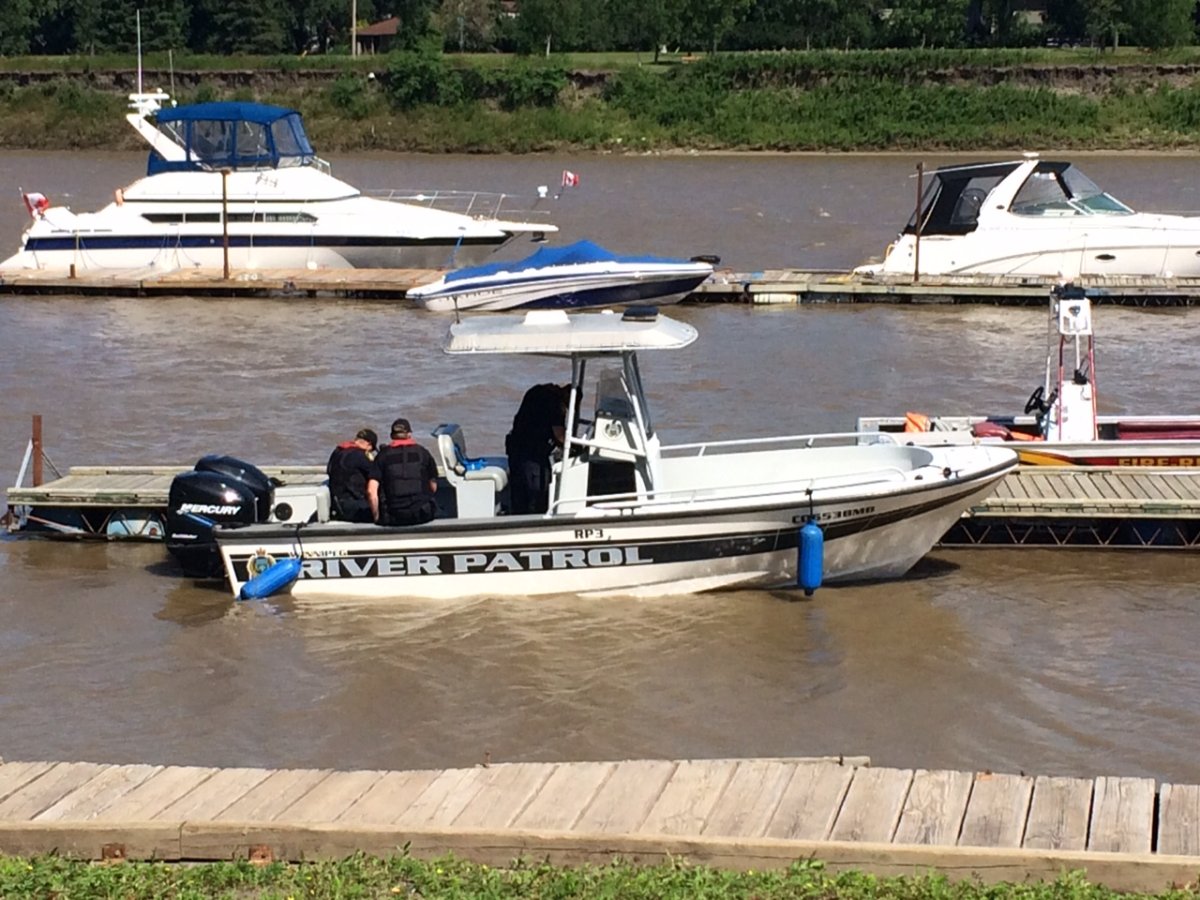The image captures a bustling scene on a muddy river, enveloped by grassy banks on both sides. In the foreground, a wooden dock extends into the water, adjacent to a boat labeled "River Patrol," where four individuals are visible; they are dressed in black vests, pants, and hats, likely indicating some official capacity, and wear pink flotation devices around their necks. The river patrol boat appears docked, and the men are either sitting on the edge or close to the steering wheel. In the murky brown waters beside it, three more boats of varying shapes and sizes float. The boat furthest to the back left is a small white yacht with a blue top, while a smaller speedboat and another personal use boat are nearby. These latter boats are unoccupied and mostly white with black accents, except for the one with the distinct blue top piece. The chaotic but lively river scene is bracketed by the lush, green riverbanks, enhancing the image's natural setting.